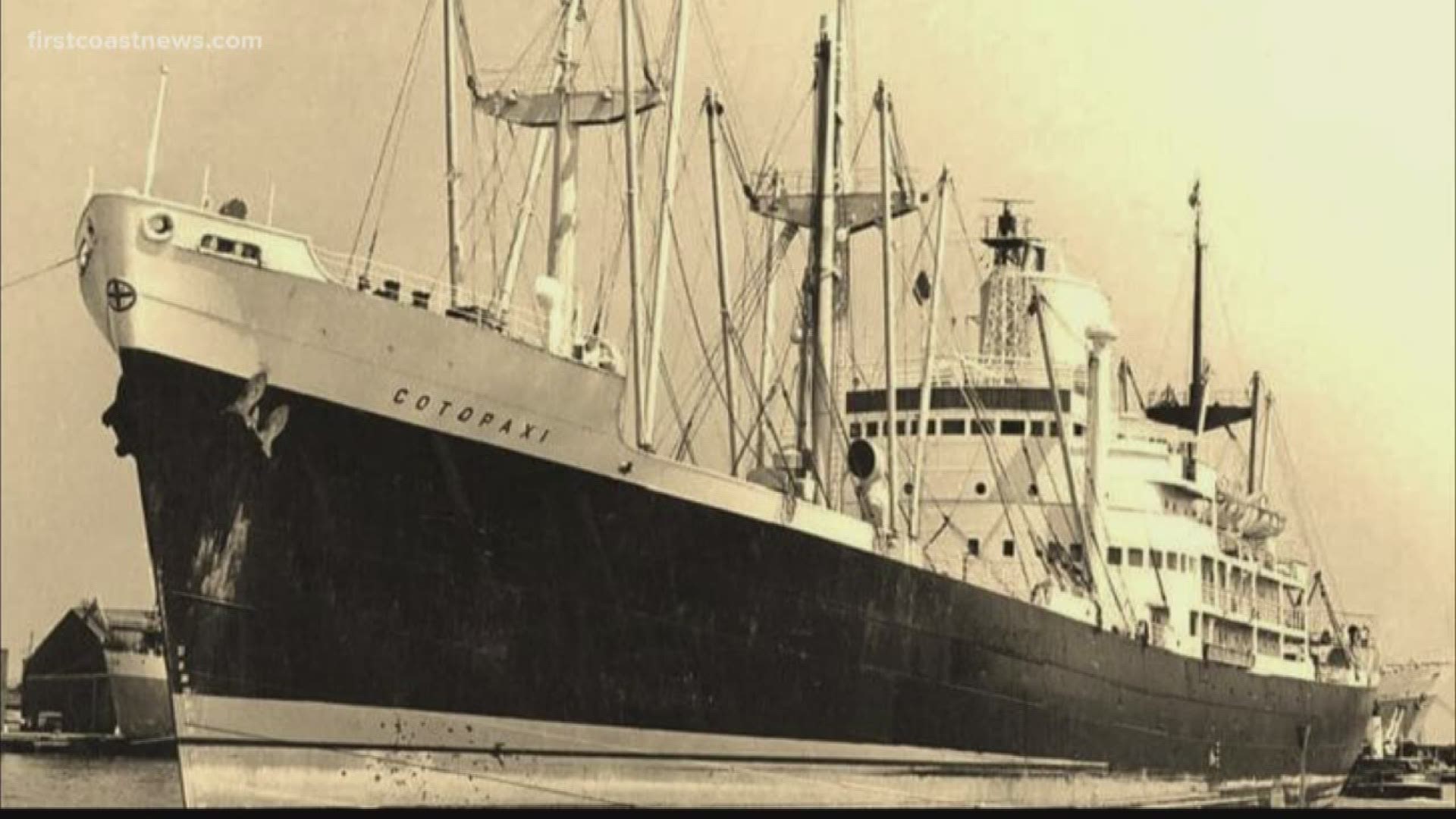This black and white photograph captures the vessel Kotopaxi, a mid-20th century steamship, docked in a harbor. The image, tinged with antique yellow tones, is a wide horizontal rectangle showcasing the ship from a diagonal perspective, with the bow positioned to the left and the prow angled towards the lower right. The Kotopaxi features a prominent smokestack and several metal poles with ropes, suggesting its steam-powered nature rather than relying on sails. The ship appears relatively unladen, indicated by the high water line. The exterior displays a white top, black midsection, and white bottom. Behind the vessel, smaller boats and harbor structures are visible. Despite its apparent age, the photo's precise temporal origins seem to place it in the late 1950s or early 1960s. The name "Kotopaxi" is clearly legible along the side of the ship, and it appears to come from a website, though the specific source remains unnamed.